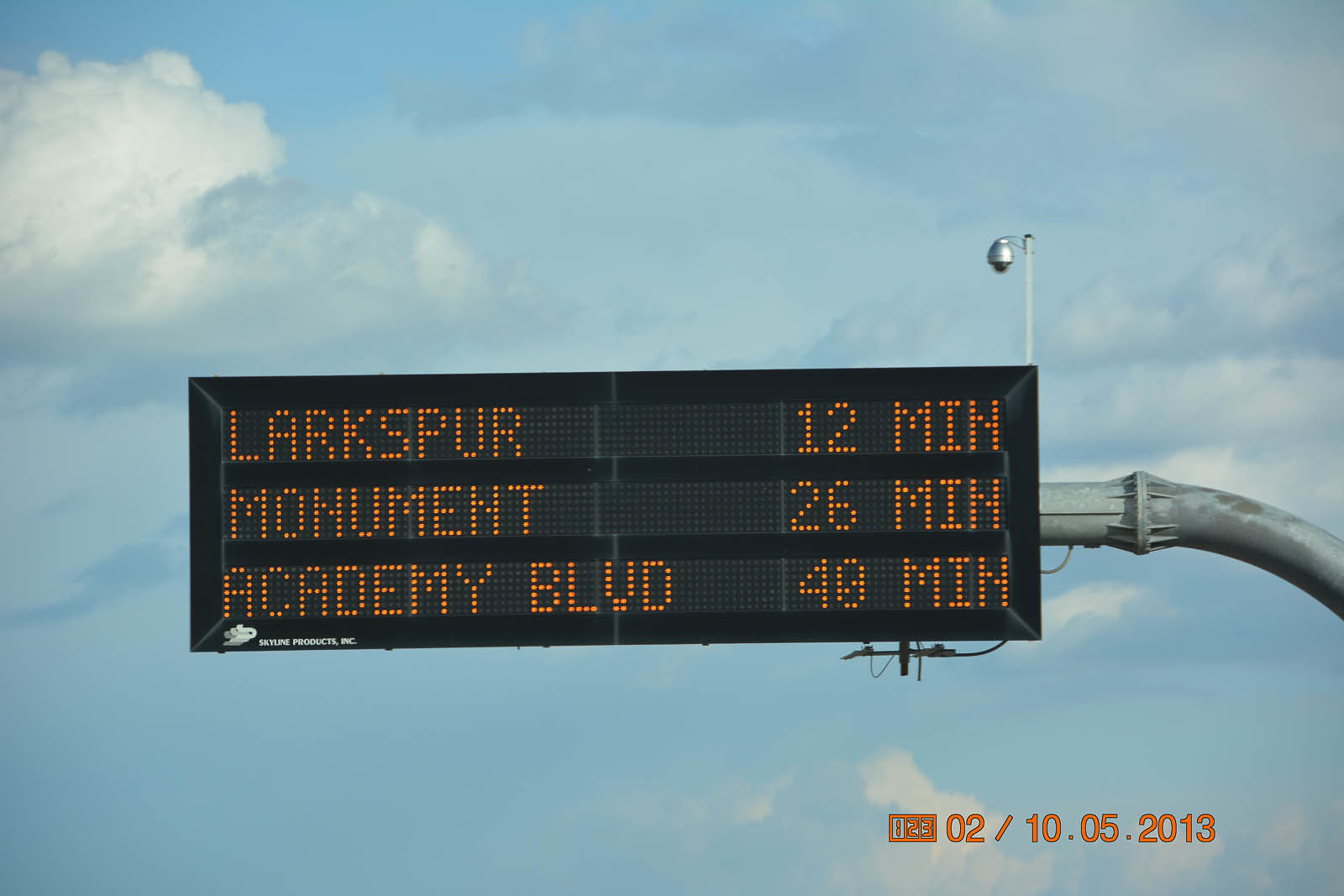This photo depicts a digital highway sign, hanging horizontally from a metallic rod against a bright midday sky, filled with patches of white and hazy clouds. The signage, displaying traffic information in orange text on a black background, has three lines: "Larkspur, 12 minutes" at the top, "Monument, 26 minutes" in the middle, and "Academy Blvd, 40 minutes" at the bottom. Each destination's name appears on the left, with corresponding travel times on the right. In the bottom right corner of the photo, a timestamp reads "02/10.05.2013, 123" in the same orange hue. The background is a seamless expanse of light blue sky, emphasizing the outdoor setting.